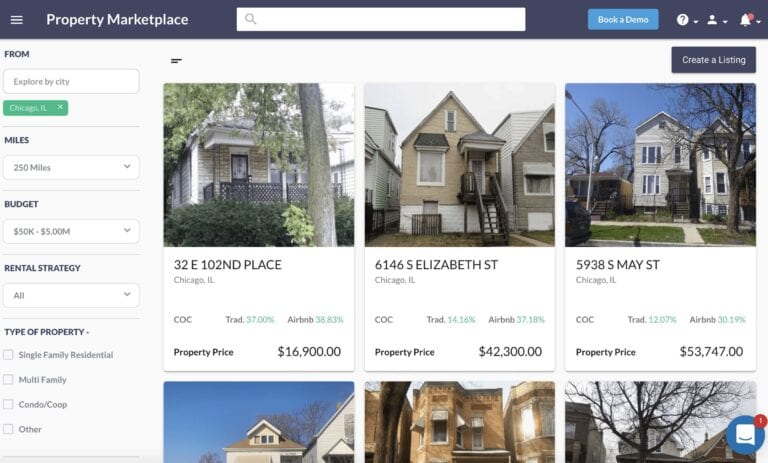A detailed screenshot captures a property marketplace interface. On the top left corner, a recognizable hamburger menu symbol is present. On the opposite side, the top right corner features several icons including 'Book a Demo,' a question mark for help, a profile icon, and a notification bell with a red dot indicating new notifications.

Prominently centered is a search bar facilitating user queries. Below the search bar, various filters are available, including options to "Explore by City," with distance parameters set at 250 miles, budget, rental strategies, and property types. Checkbox options allow selection among Single Family Residential, Multifamily, Condo/COOP, and Other types of properties.

At the top right of the interface, a blue rectangular button labeled "Create a Listing" in white text stands out. The screen also displays a list of properties with their corresponding details:

1. **32 E. 102nd Place, Chicago, Illinois** - Property Price: $16,900
2. **6146 S. Elizabeth Street, Chicago, Illinois** - Property Price: $42,300
3. **5938 May Street, Chicago, Illinois** - Property Price: $53,747

This detailed view emphasizes the functionality and layout of the property marketplace platform.